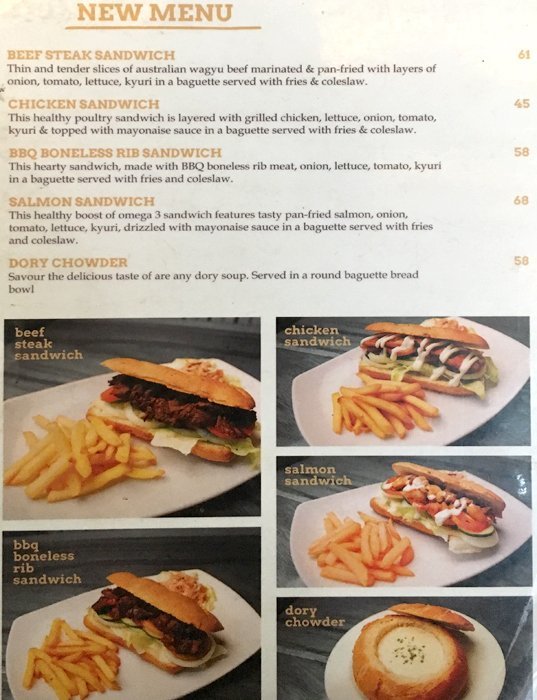This full-color menu page features a clean white background and showcases five vibrant photographs of various dishes. At the top of the placard, "New Menu" is elegantly written in gold, followed by the name and description of each dish in smaller gold and black text, respectively.

The dishes include:
1. A juicy beef steak sandwich, clearly labeled as menu item #61.
2. A hearty chicken sandwich, presumably grilled to perfection.
3. A savory barbecue boneless rib sandwich, dripping with flavor.
4. A fresh and enticing salmon sandwich, likely seared or smoked.
5. A rich and creamy dory chowder, hinting at a comforting soup.

The menu page suggests a warm, mid-level family restaurant atmosphere, emphasizing approachable and satisfying meals without any pretentious or extravagant touches.